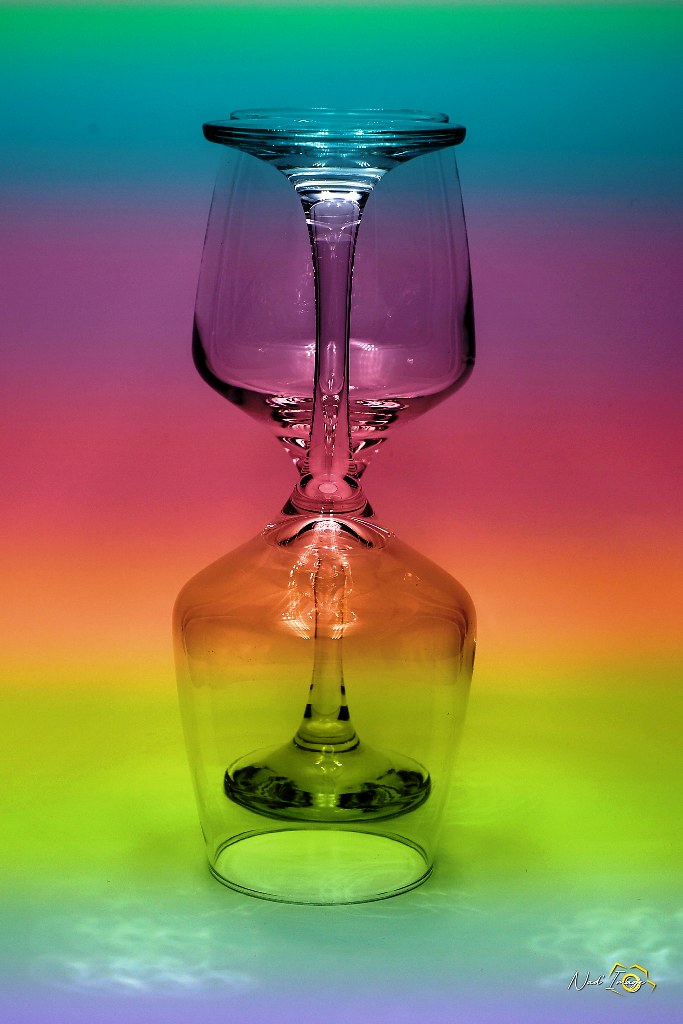This vertical, rectangular poster showcases a photograph of two wine glasses arranged in a unique, stylized manner. The glass in the foreground is upside down, with its drinking part on the ground and its stem pointing upward, while the second glass behind it stands upright. These overlapping glasses, being transparent, allow the viewer to see the stems through the bowls. The background features a gradient rainbow of horizontal sections starting from the top with bright green, followed by blue, purple, pink, coral red, orange-yellow, lime green, and ending with light sea blue, and another purple band at the bottom. The rainbow hues blend together, giving the image a dynamic yet harmonious feel. There is a small, unreadable artist's watermark or logo located in the bottom right corner.